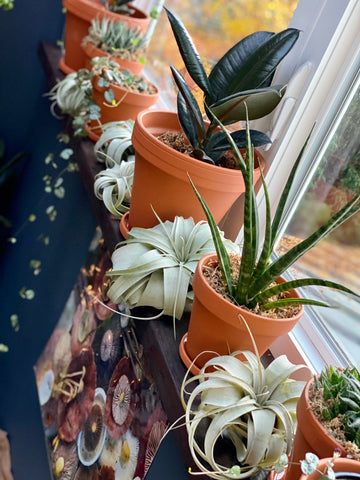The photograph captures a vibrant windowsill, which serves as an impromptu shelf for a variety of potted plants. The angle of the shot is from above, at roughly a 30-degree angle, making it appear as though the photographer is looking down on the scene. The windowsill, wide and black in color, is perfectly adequate to accommodate numerous potted plants arranged across its surface. The white-framed window on the right side of the image provides a luminous backdrop, showcasing a glimpse of the green outdoors, possibly featuring a stretch of road. The window appears to be closed.

The wall to the left of the window is painted a light blue and hosts a hanging picture, which seems to depict some form of plant life. The plant pots themselves are brown, and amidst them are interspersed distinctive white plants, adding a unique contrast to the overall display. Among the plants, an aloe vera is identifiable, contributing to the lush and varied greenery on the windowsill.